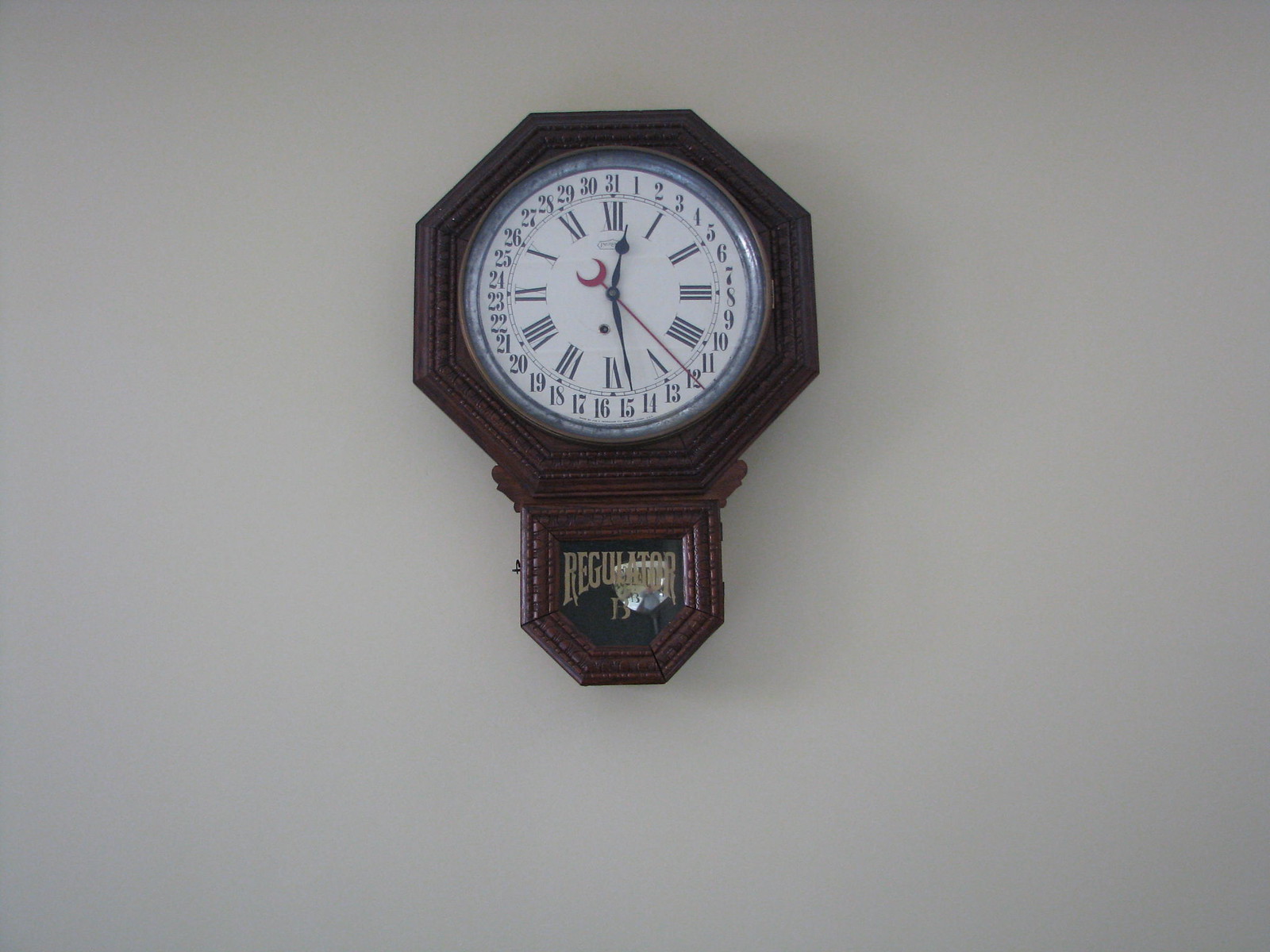This image showcases a beautifully crafted wooden grandfather-style wall clock. The clock prominently features an octagonal top with a large, round white face bordered by a thin blue ring. The face is adorned with Roman numerals at its center and regular Arabic numerals around the periphery. Above the 12 o'clock position, the number 31 is displayed, likely indicating the date. A notable feature is a large red hand with a crescent moon tip, pointing exactly at 12. The classic hour and minute hands are black; the hour hand has a spade-shaped tip and indicates the time as approximately 12:29.

Below the clock face, a wooden section with a glass front houses a circular chime mechanism. The word "REGULATOR" is inscribed in yellow above the chime, with an unreadable number situated below. The entire clock contrasts elegantly against the plain white wall it rests upon.